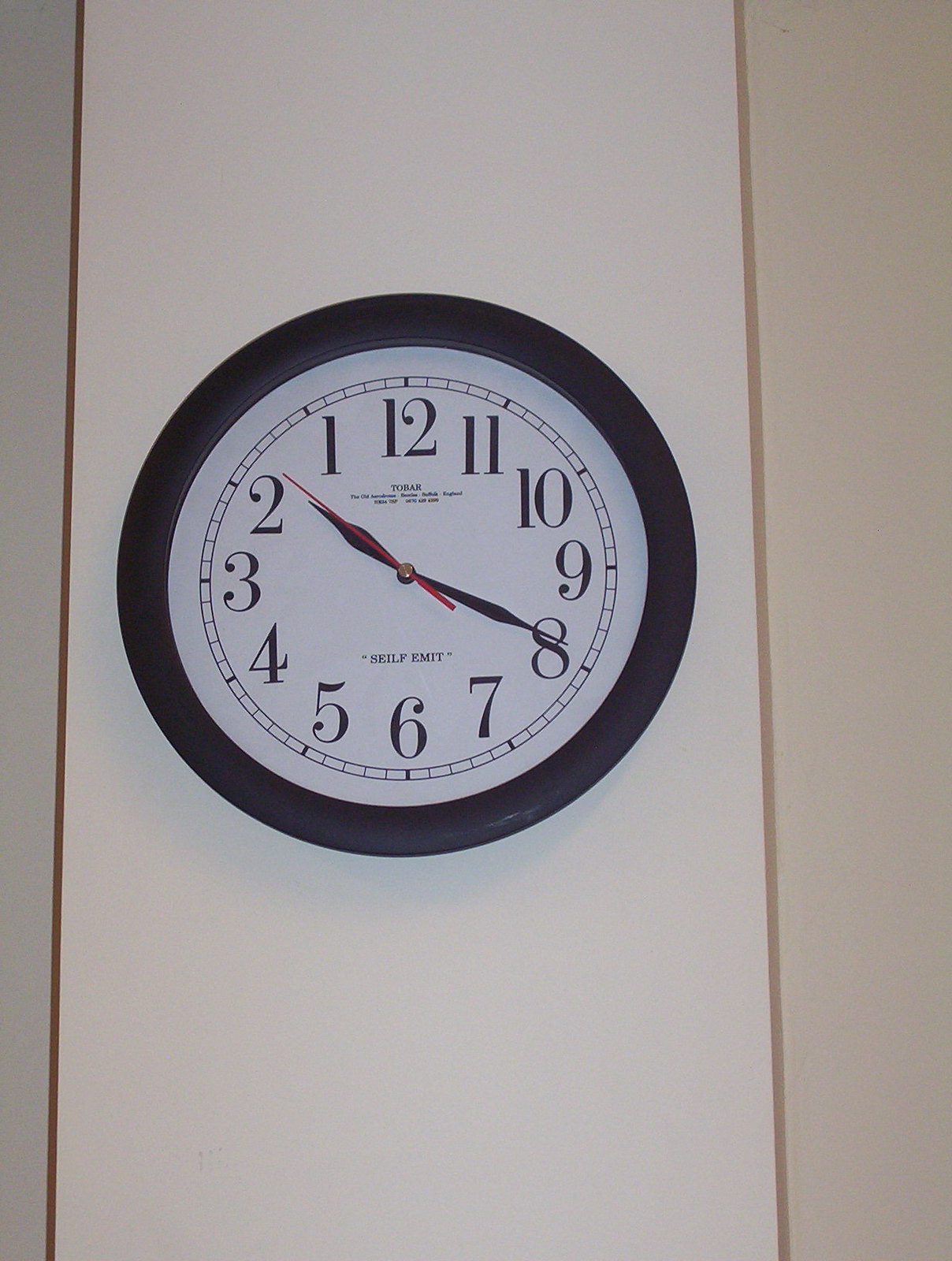This photograph features a black clock mounted on a pristine white wall. The clock face itself is white and is encircled by two subtle gold lines running down the wall, adding a touch of elegance to the minimalist setting. The clock, with a plasticky appearance, is equipped with three hands: two black for hours and minutes, and one red for seconds. Uniquely, the numbering on the clock is in reverse order, starting at 12 and ending at 1, creating an unconventional and eye-catching design.

Beneath the number 12, there is some small black font, though the details are not easily discernible. The clock face is marked with black dash marks indicating the minutes. The photograph also captures a slight light glare reflecting off both the white wall and the clock's surface, contributing to the clarity and sharpness of the image. The overall quality of the photograph is exceptionally high, showcasing every detail with crystal clear precision.